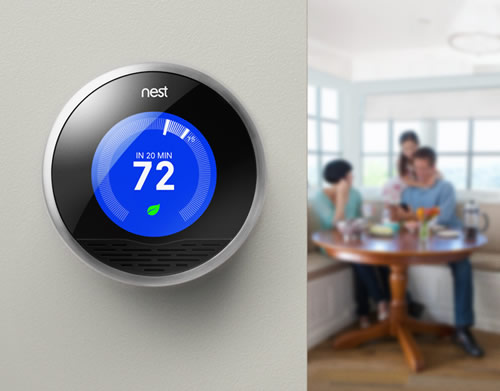In this advertisement image for a Nest thermostat system, we see a meticulously designed Nest thermostat mounted on a white wall on the left side of the picture. The thermostat boasts a sleek stainless steel or silver plastic frame encasing it. Inside this frame, there's a glossy black ring encircling the device's digital interface. The center of the thermostat features a blue spot with a digital gauge displaying a temperature of 72 degrees in clear white numerals. The word 'Nest' is prominently displayed in white at the top of the thermostat.

The right side of the image showcases a blurred yet cozy family scene in a kitchen. A family sits around a brown round table, seemingly enjoying dinner. The mother, positioned on the left, is dressed in a green shirt and has black hair. Opposite her, the father is clad in blue jeans, black boots, and a blue shirt. A small child, standing behind the father and affectionately hugging his neck, is dressed in brown and also has black hair. The kitchen setting is bright with white cabinets and a white ceiling, adding to the overall warm and inviting atmosphere of the scene.